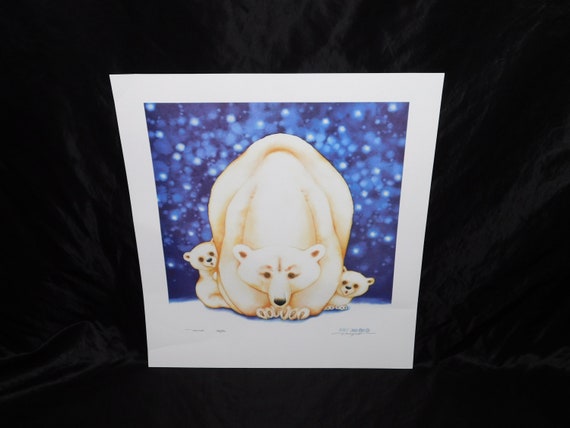The image in question appears to be an art print styled like a Polaroid photo. It features a family of animated polar bears—presumably a mother bear with two cubs—situated on a pristine, white snowy surface. The mother bear, centrally positioned and significantly larger than the cubs, is depicted with her head down and her front paws touching the ground. The cubs are positioned to the left and right of her, near her paws. The background behind the bears is a deep, sparkling blue, resembling a starry night sky, with various shades of blue and white dots scattered across it. The square image is framed by a white border, which is thin on the left, right, and top edges, and slightly thicker at the bottom, reminiscent of classic Polaroid photographs. The overall image is bright and clear, with no visible text or letters, and the art print stands out against a black backdrop that envelops part of the top and left sides.